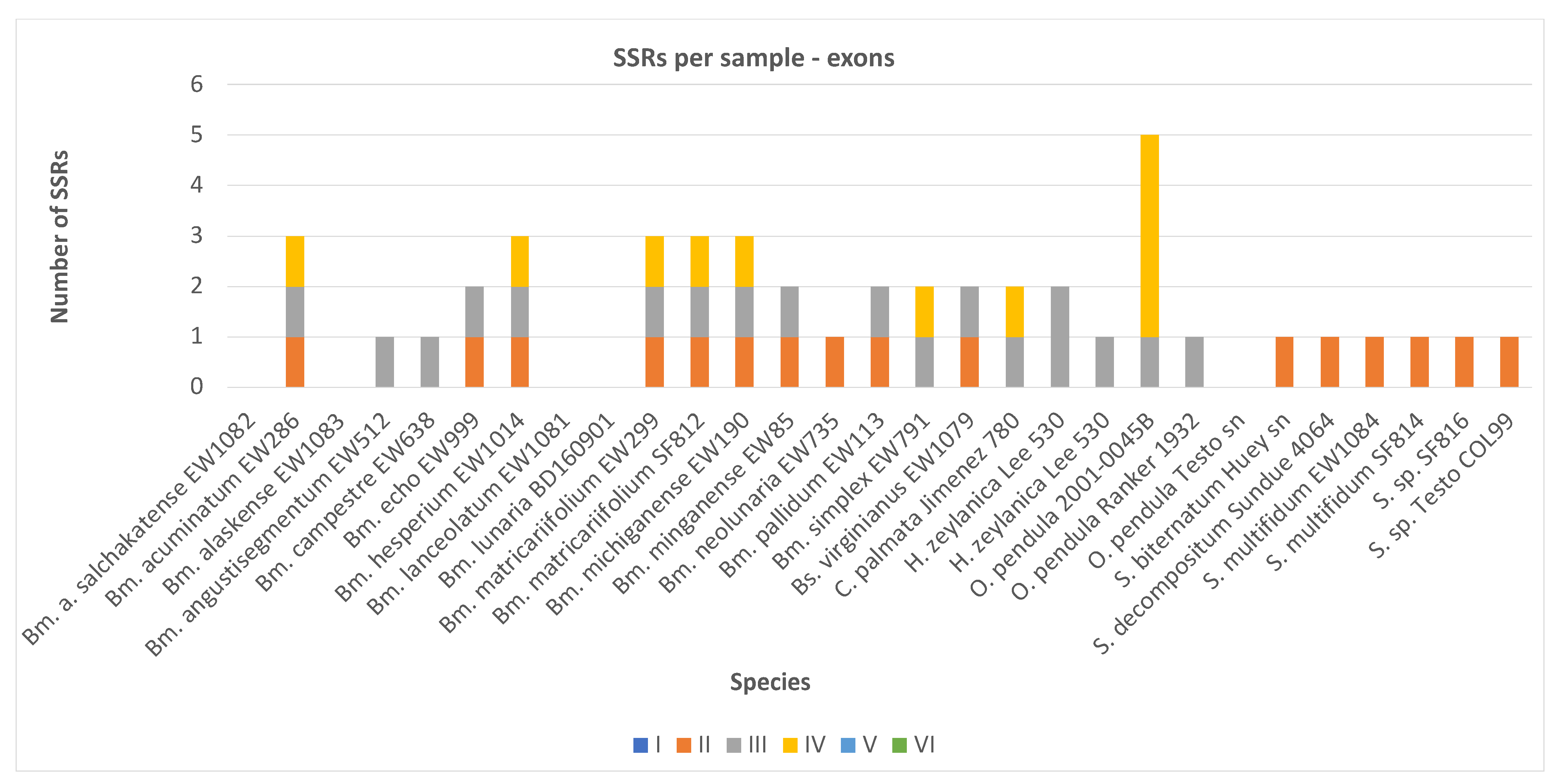The image is a highly detailed bar graph titled "SSRs per sample - Exons." The y-axis represents the "Number of SSRs," scaled from 0 to 6, while the x-axis indicates various species labeled with abbreviations like "bm, a, sal, ch, ak, te, n, se." There are 29 different species in total. Each bar in the graph is divided into colored segments: blue for Roman numeral I, orange for II, gray for III, yellow for IV, light blue for V, and green for VI. The legend under the x-axis clarifies these colors. The bars range from 0 to 5 in height, with the majority falling between 0 and 3. Each color segment within the bars represents distinct species categories and their respective SSRs, indicating a detailed comparison across various exons, possibly for botanical research. Species names such as Salcatracatens, Acuminatum, Alaskans, Angustisegmatum, Campestra, Echo, Hesperitum, and Lanceolatum are included, highlighting the diverse data set.